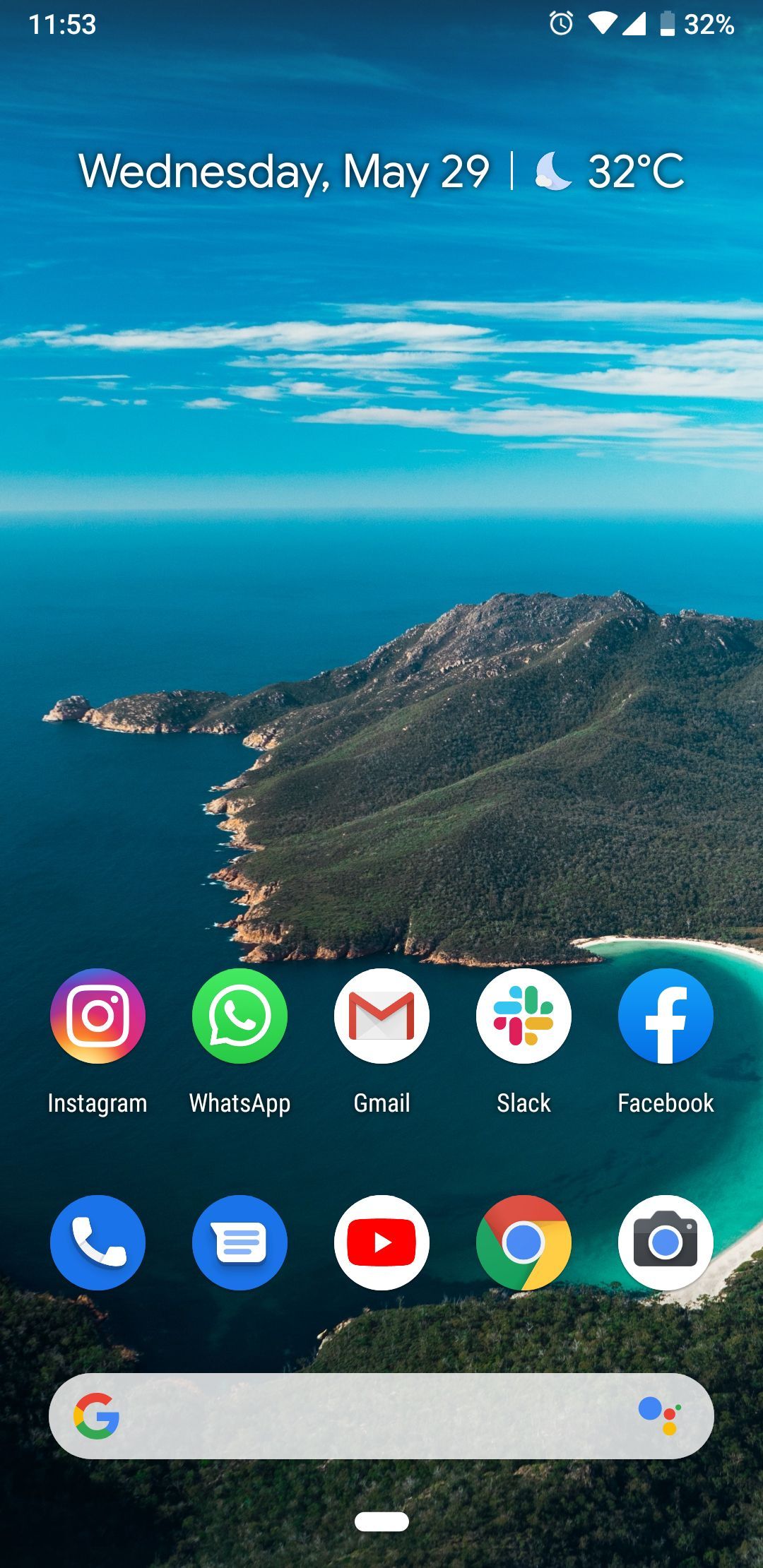A stunning aerial view adorns the home screen of an Android device, showcasing a picturesque tropical island. The coastline cradles a serene bay filled with light green and teal waters, surrounded by sandy shores. Beyond the bay, the scenery transforms into rocky shorelines and majestic cliffs, all blanketed in lush greenery. The sky is adorned with light, fluffy clouds drifting in the distance, accented by wisps of cirrus clouds high above.

In the top left corner, the time is displayed at 11:53. Adjacent to it on the right are icons indicating full Wi-Fi signal, a clock, and a battery level at 32%. Below this, centered in white text, the date reads "Wednesday, May 29th," accompanied by the temperature of 32 degrees Celsius.

The interface is organized with two rows of icons at the bottom. The upper row includes frequently used apps: Instagram, WhatsApp, Gmail, Slack, and Facebook, all labeled with their names beneath them. The lower row comprises essential icons: phone, messaging, YouTube, Chrome, and camera, each identifiable sans labels. At the very bottom, a Google search bar invites inquiries, completing the home screen layout.